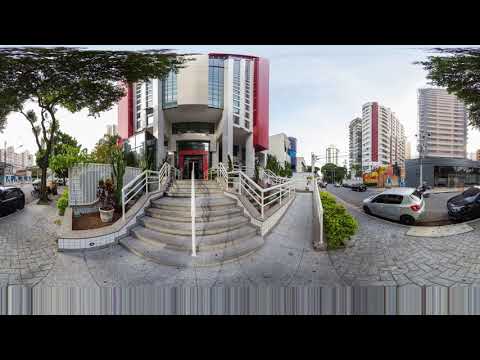In this 360-degree view image, we see a central stairway leading up to a building, likely in a major city area. The stairway is flanked by railings and surrounded by a stone pathway and concrete walkway. The building remains ambiguous, potentially serving as either an administrative facility or an apartment complex. This outdoor scene, captured on a sunny day with clear blue skies, shows no visible people or animals. Flanking the staircase are various plants and shrubs, adding a touch of greenery. In the distance, several reasonably tall buildings are visible along with a few parked cars on either side of the roadway. The borders of the image have a solid black edge, and the overall color palette includes hues of black, gray, red, tan, green, yellow, orange, and light blue. The photo appears slightly distorted, possibly due to the lens used, and is taken in broad daylight, somewhere likely downtown.